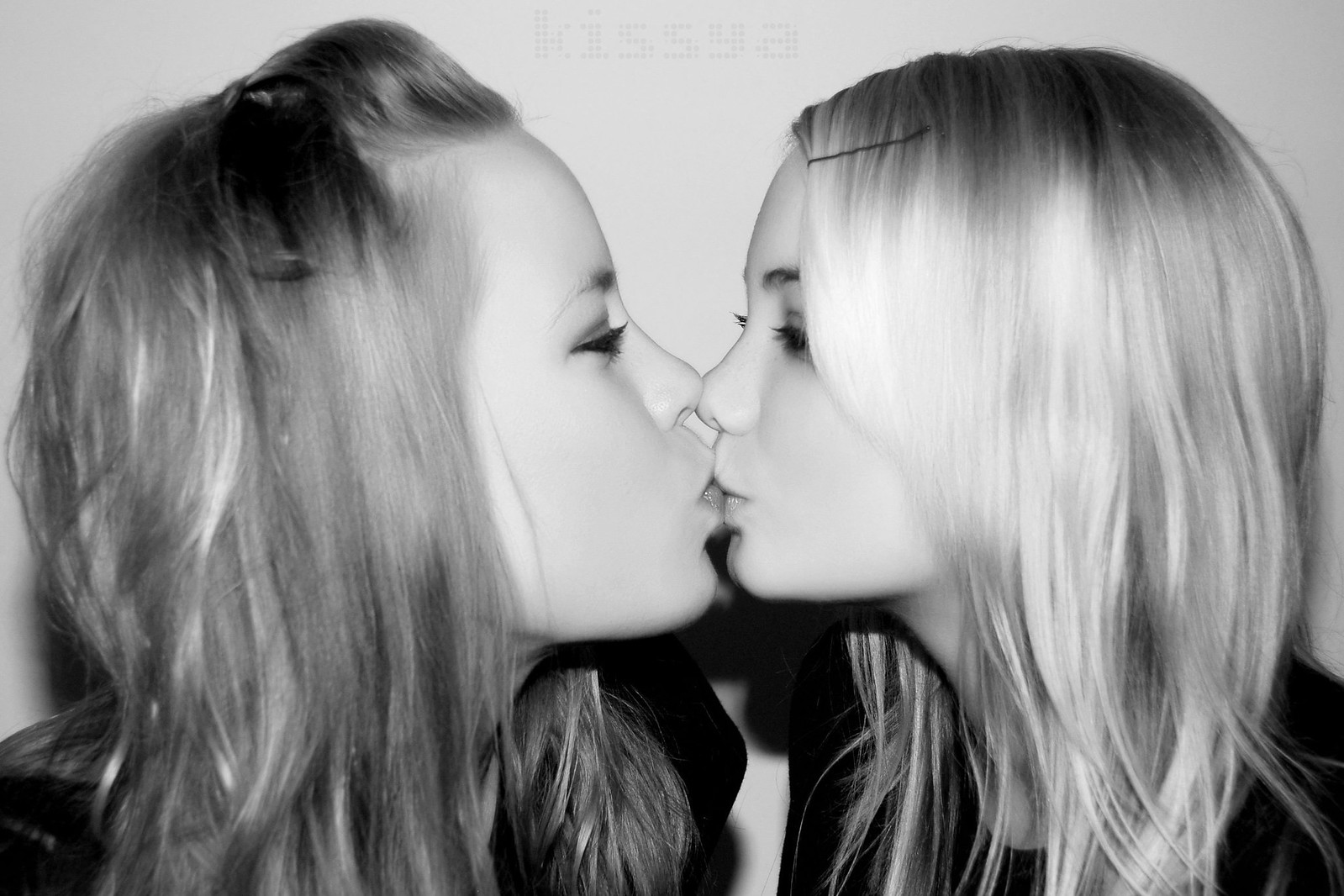The black and white image features two young, blonde-haired girls with straight hair, who appear similar in their facial features. They are depicted kissing, with their noses and lips touching, and they are facing each other in a playful, possibly staged manner. They are both white and wearing black clothing, which looks like it could be sweaters or jackets, hinting at a colder season. Their hair is styled with accessories; the girl on the right has a bobby pin, while the girl on the left has a hair clip securing some of her hair at the top. Both girls are wearing mascara, and the one on the left has slightly more eyeshadow. The background is white and greyish, with a text at the top spelled out in a grey, gridded dot pattern reading "K-I-S-S-Y-A." This image may be considered offensive to some viewers due to its content.